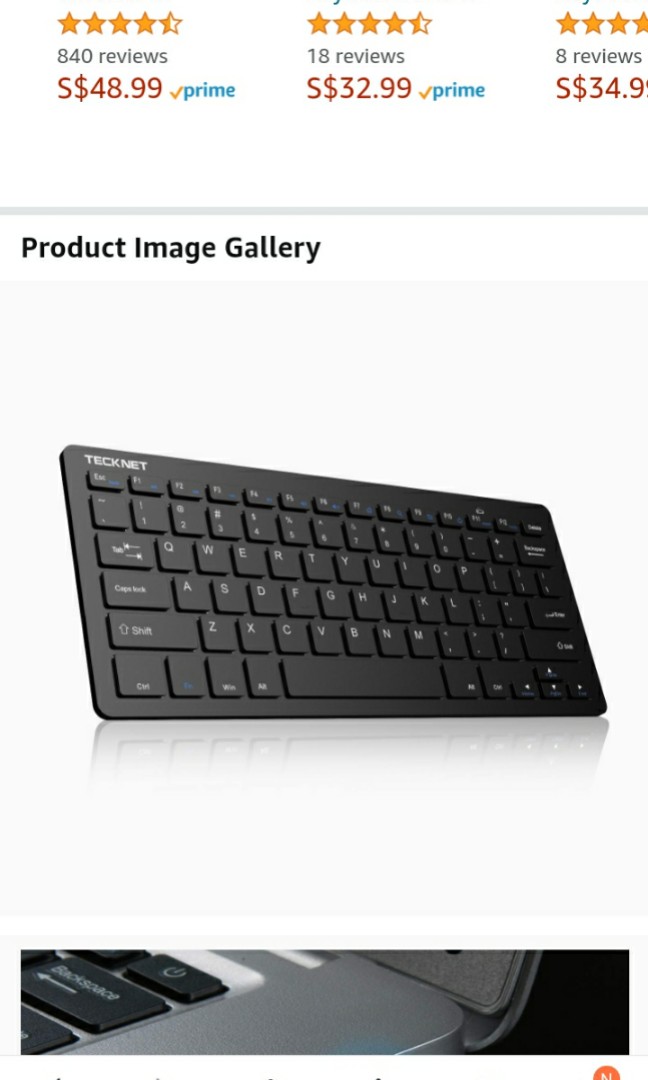The image features a product gallery for a keyboard against a white background. At the top, a review section shows four and a half yellow stars, with the remaining portion of the fifth star unfilled. Below the stars, "840 reviews" is written in black font. The price is listed in red as S$48.99, accompanied by the Amazon Prime logo, which includes a yellow check mark and the word "Prime" in blue letters.

The next row showcases another product review with four and a half stars and "18 reviews" in black font underneath. The price for this product is S$32.99 in red, with the Amazon Prime logo next to it. There is a third product in this row, which is partially cut off in the image. It displays four stars, "8 reviews" in gray font, and a price of S$34.99 in red font.

Underneath this section is a gray line, followed by the text "Product Image Gallery" in black font on the left. The main product image shows a black keyboard named "TechNet" inscribed in white font on the top right corner. The keyboard casts a slight shadow at its base. Below this, there is a close-up view of a laptop with a gray side and a black background. A half-circular orange logo with the letter "N" in white font is visible on the laptop.